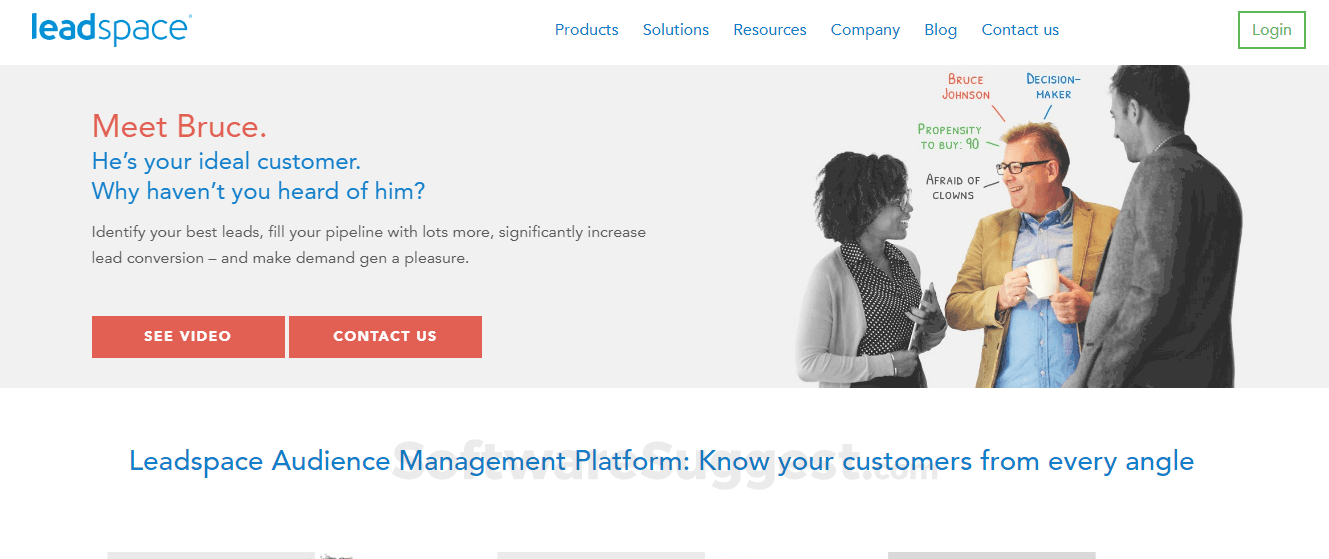Here is a concise and detailed caption for the image:

---

Screenshot of a web page with a predominantly white background. The top-left corner features the word "lead" in bold turquoise, followed by the word "space" in regular turquoise font. To the right, there is a navigation bar with clickable blue links labeled "Product," "Solutions," "Resources," "Company," "Blog," and "Contact Us." A green rectangle with the word "Login" inside is also present.

Below the navigation bar is a light gray rectangle. On its left side, the text "Meet Bruce" appears in red letters. Beside this, a blue sentence reads, "He's your ideal customer. Why haven't you heard of him?" Below this, a smaller black text is slightly difficult to decipher. Within the gray rectangle are two orange buttons: one labeled "See Video" and the other "Contact Us."

On the right side of this gray rectangle, there is a large image. It features three individuals: a woman in black and white looking to the right, a man in black and white looking to the left, and a man in color positioned centrally. The central man, with blonde short hair and glasses, is wearing a suede jacket over a blue shirt. Surrounding his head are various colorful elements.

---